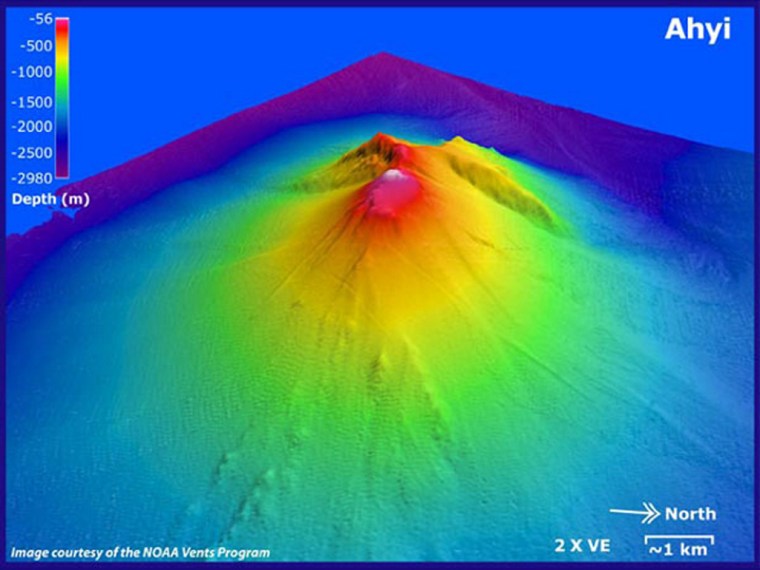This image is a detailed digital representation of an underwater volcano, created using a program that visualizes heat signals as depth indicators. The rectangular image features a vibrant and colorful chart where colors ranging from red to purple denote varying depths, not temperatures. The shallowest depth, marked in red, is negative 56, while the deepest, represented in purple, reaches up to 2,980. The top left corner includes a depth scale, showing a gradient from red at the highest point to purple at the lowest. The visual forms a towering formation resembling a volcano, colored blue at the base, transitioning through green and yellow, and culminating in red and pink near the peak. A thin dark blue border frames the entire image. The top right bears the label "AHYI," and the image credit at the bottom left reads "Image Courtesy of the NOAA Vents Program." Additional notes on the bottom right provide further context about the size and location of the volcano.